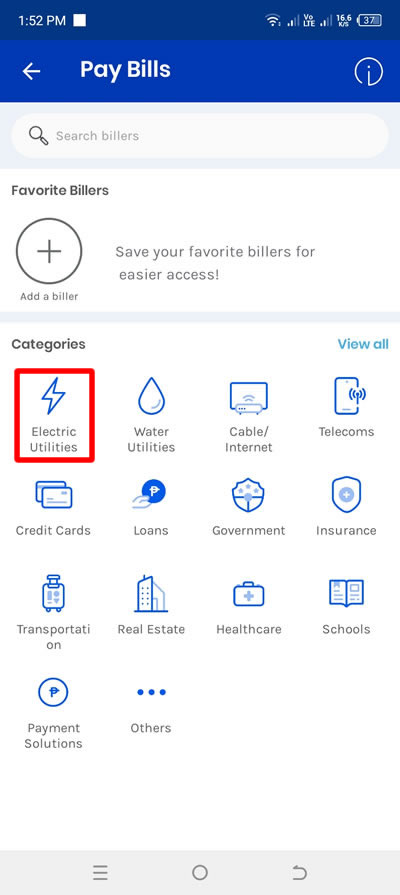A detailed screenshot of a mobile bill payment interface displaying various bill categories and navigation options. The time displayed on the top-left corner is 1:52 PM. At the top of the screen, within a blue header bar, there is a left-pointing white arrow and an eye icon enclosed in a white circle. The text "Pay Bills" is prominently featured in this header area. 

Below the blue header, there is an empty search field labeled "Search Billers." Underneath, the section titled "Favorite Billers" includes a large plus icon accompanied by the text "Add a Biller" and a subtitle that reads "Save your favorite billers for easier access."

The main section of the interface is organized into categories, each represented by a corresponding icon:

- **Electric Utilities:** Represented by a lightning bolt icon, which is highlighted by a red box.
- **Water Utilities:** Denoted by a water droplet icon.
- **Cable/Internet:** 
- **Telecoms:** 
- **Credit Cards:** 
- **Loans:** 
- **Government:** 
- **Insurance:** Represented by a shield icon.
- **Transportation:** 
- **Real Estate:** 
- **Healthcare:** 
- **Schools:** 
- **Payment Solutions:** 
- **Others:** 

At the top of the categories section, there is an option "View All" in blue text, allowing users to see all categories at once. 

The bottom portion of the screenshot shows the mobile phone’s navigation bar with common icons such as a circle, three horizontal lines, and a left-pointing arrow, indicating standard navigation controls.